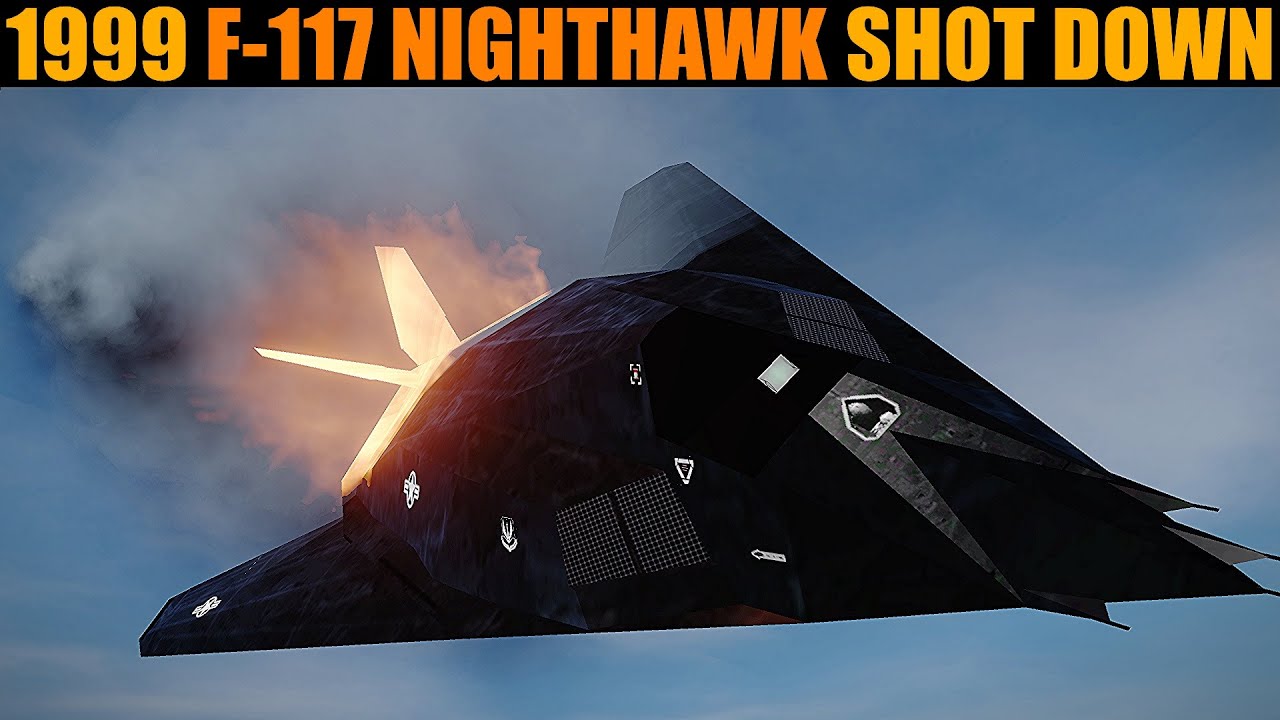This rectangular image, approximately 5 to 6 inches wide and 3 inches high, features a vivid scene set against a blue sky with wispy clouds. Dominating the top section is a black header, about half an inch deep, emblazoned with large, all-capital letters in striking yellow and orange. The text reads "1999 F-117 Nighthawk SHOT DOWN," with "1999" and "SHOT DOWN" in yellow, and "F-117 Nighthawk" in orange. 

The central focus of the image is a stylized illustration of a stealth aircraft, mainly black in color with grey accents and silver stickers. The aircraft, almost triangular in shape with V-shaped tail fins, is depicted mid-flight and facing towards the right. The scene dramatically captures the aircraft in apparent distress, with bright flames and thick, dark smoke emanating from its rear. The fiery glow at the back starkly contrasts with the stealthy design of the plane. The details, such as its cockpit windows and the malfunctioning engines, are prominently visible, emphasizing the dire situation.